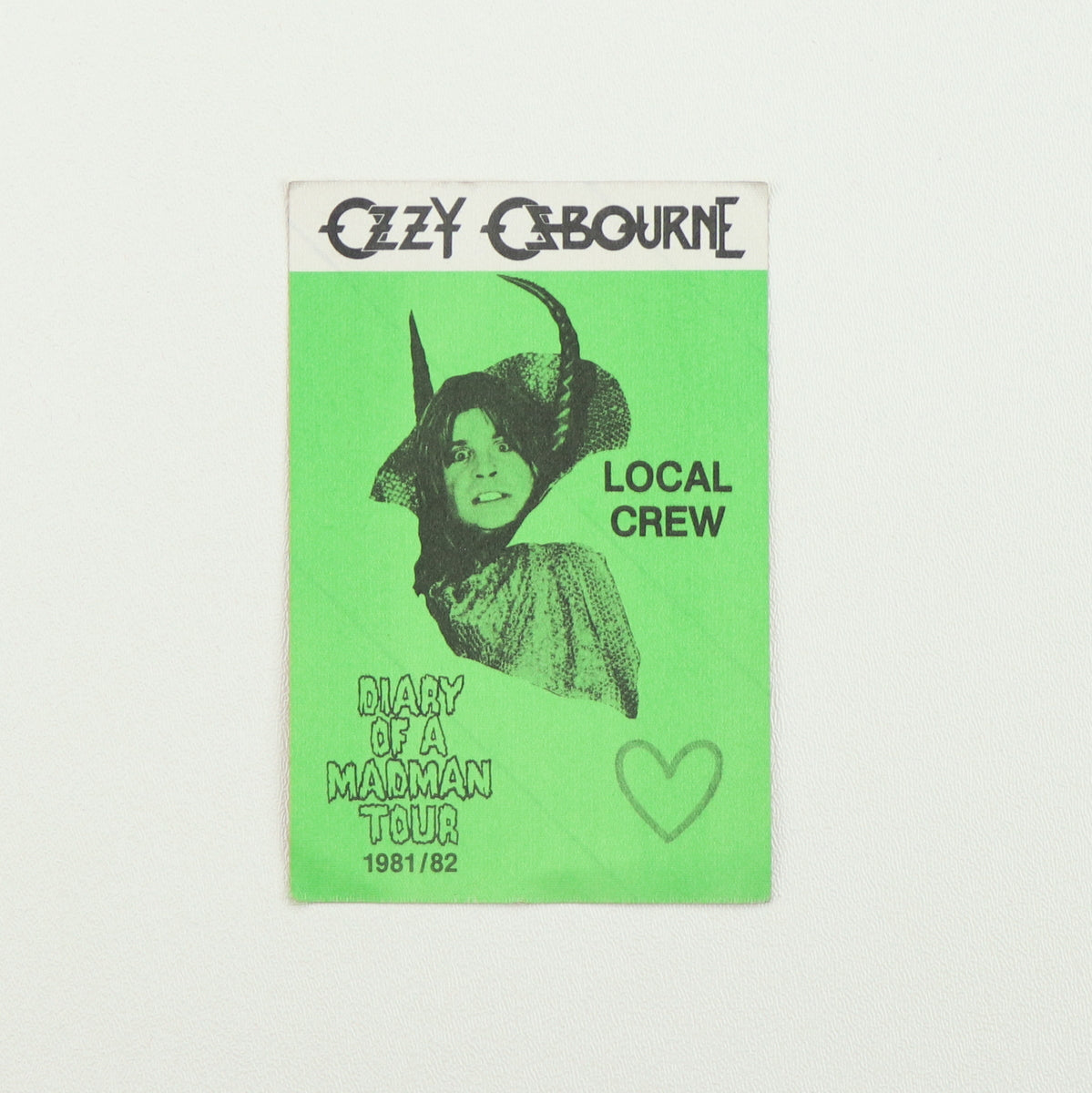This image features a vintage Ozzy Osbourne concert flyer against a plain gray background. The top of the flyer has a white stripe with "Ozzy Osbourne" printed in black letters. The majority of the flyer is a vivid mint green color, and centrally displayed is a black and white depiction of Ozzy Osbourne, adorned with devil horns and a cape, giving a panicked expression. His long, shaggy hair adds to the chaotic vibe, and he is connected to a disembodied tube. The text "Local Crew" is positioned next to the image. At the bottom left-hand side, it reads "Diary of a Madman Tour 1981-82," and a light gray heart decorates the bottom right corner.